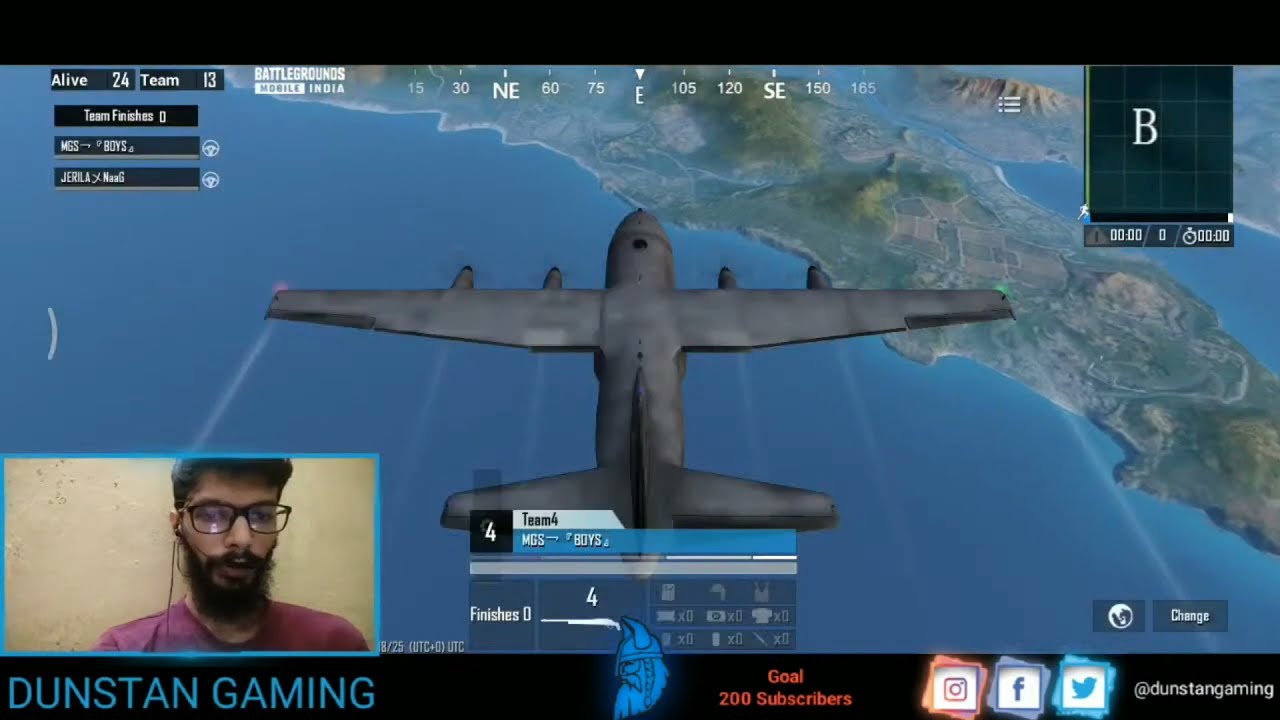The image is an animated still frame from a video game, featuring a large, gray military-style airplane flying over the ocean with a finger-shaped island in the background. Viewed from a top-down, third-person perspective, the airplane's wings are extended with green and red lights on opposite ends, and motion-blurred propellers are visible near each wing. The island below is a mix of green and brown with hilly areas, while the ocean occupies the rest of the scene.

The screen has multiple overlays. At the top left corner, there is text indicating "Battlegrounds Mobile India" and gameplay stats: "Alive 24, Team 13, Team Finish 0." A navigation compass shows the plane flying east, with northeast and southeast markers. A grid map with a "B" marker and a timer reading "00:00" are located at the top right.

The bottom of the screen features a black rectangle displaying the message "Goal: 200 subscribers" in orange, flanked by logos for Instagram, Facebook, and Twitter in white squares. Below this is the title "Dunstan Gaming" in blue font, accompanied by an at symbol (@Dustan Gaming). A logo of a cartoonish Viking head with horned helmet and large beard is adjacent to the title. 

In the lower-left corner, a picture-in-picture frame shows a Middle Eastern or Indian man with black hair and glasses, wearing a crimson red t-shirt and a beard, likely the game's streamer. Below his image, "Dunstan Gaming" is inscribed in blue font.